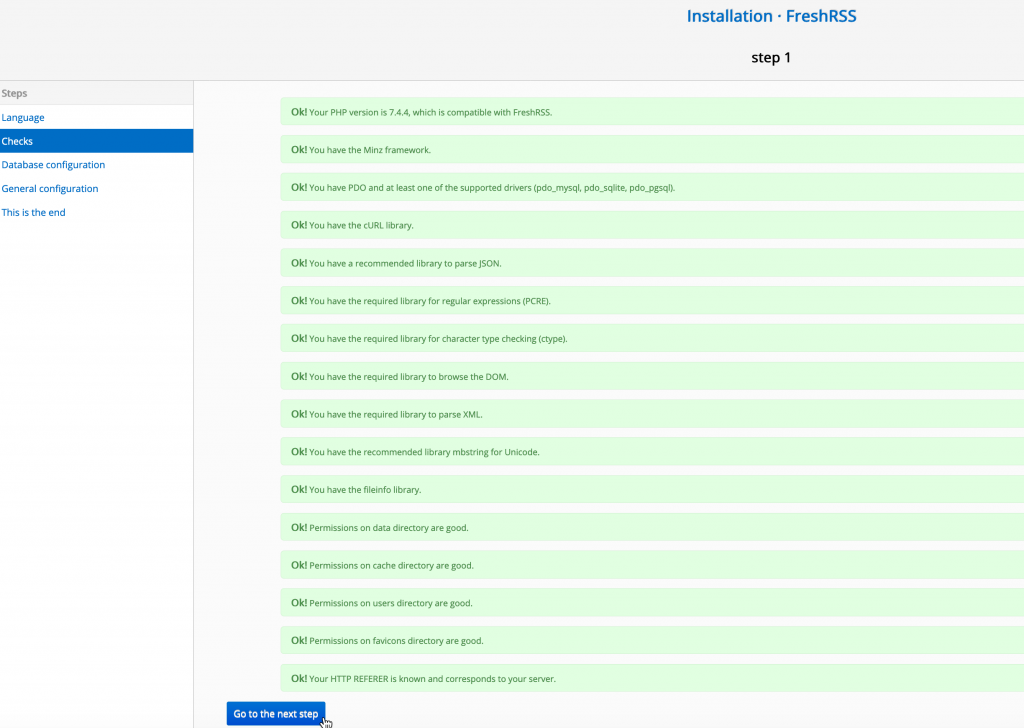The image captures a step-by-step installation process for FreshRSS, a self-hosted RSS feed aggregator. At the top of the interface, the user is at the 'Checks' stage, indicated by a highlighted blue section on the progress bar, which lists the stages as 'Language', 'Checks', 'Database Configuration', and 'General Configuration'. The installation screen confirms various system requirements in a sequence of green dialog boxes. These include the PHP version 7.4.4 compatibility, the presence of the Mens framework, and the PDO extension, among others. Altogether, there appear to be around 15 system checks, each validated with an "OK" in green boxes. Once all checks are confirmed, the user can proceed to the next step by clicking a prominently featured blue button labeled 'Next Step'. The background of the page is a light gray, contrasting with the white content area. The column on the right, displaying the language options and installation steps, is also white with blue textual elements. The cursor is seen hovering near the navigation button.